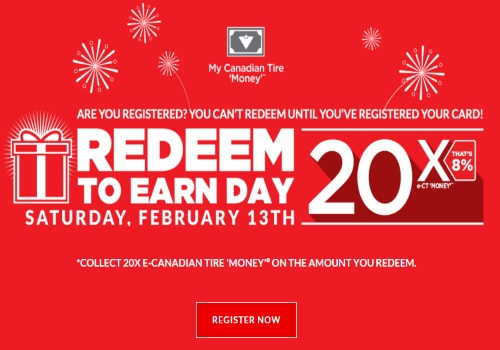Promotional Advertisement for Redeem to Earn Day at Canadian Tire

The image is a vibrant promotional advertisement for Canadian Tire's Redeem to Earn Day. The background is strikingly bright red with complementary white and red accents. At the top center of the image, there's a small rectangular graphic featuring a heart icon alongside the text "MyCanadianTireMoney". This section boldly asks, "Are you registered? You can't redeem until you've registered your card."

The main event is announced prominently: "Redeem to Earn Day, Saturday, February 13th." Beneath this, large text highlights the offer, "20 times eCanadianTireMoney," which translates to an 8% reward on the amount redeemed.

Adding a sense of urgency and action is a red "Register Now" button prominently displayed below the offer details. The surrounding graphic elements imitate fireworks bursting, injecting a festive and celebratory feel into the design.

Overall, the advertisement is designed to be visually stimulating with its predominantly red color scheme. Despite the heavy use of red, which could be seen as overwhelming, the design achieves its goal of catching the viewer's attention and conveying the excitement of the promotional event.